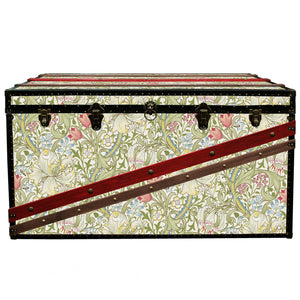This image depicts a computer-generated, classic-style steamer trunk with a distinctive, William Morris-inspired floral pattern featuring pink tulips, white flowers, and green abstract plant lines. The trunk, primarily black with black metal accents and clip locks, has a contemporary twist with diagonal decorative elements. One prominent red wood piece adorned with little brass buttons and a brown wood piece with gold buttons span from the bottom left to the top right of the trunk. The trunk’s lid has additional lines: one bright red line going from the left to the top center and several horizontal indentations consistent with traditional designs, giving it a contemporary yet vintage aesthetic.